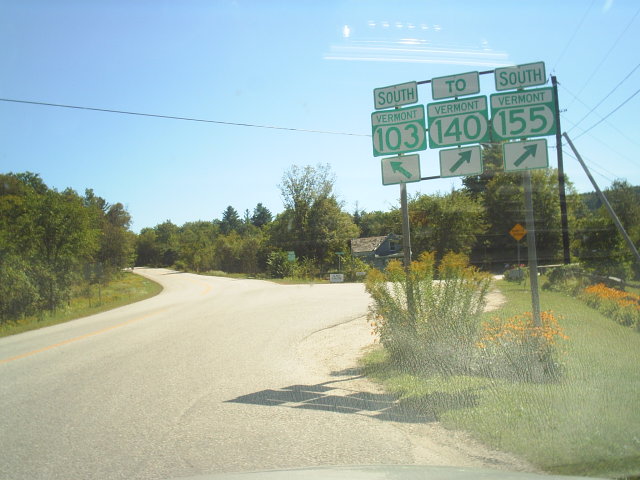The image captures an outdoor scene photographed from the middle of a dirt road, which splits into a V shape, extending left and right. The photo, taken with an older camera, has a filtered look, adding a nostalgic feel. In the background, a clear blue sky and a line of trees frame an older-looking house situated at the split of the road. Prominently placed near the center of the shot is a sign with multiple directions: "South Vermont 103" with an arrow pointing left (northwest), "To Vermont 140" pointing right (northeast), and "South Vermont 155" also pointing to the right (northeast). Adding to the rustic charm, tall weeds and yellow flowers grow at the base of the sign, and the road surroundings consist of grass and trees, with neatly mowed ditches visible. The scene exudes a serene, almost timeless quality of a remote, wooded area.